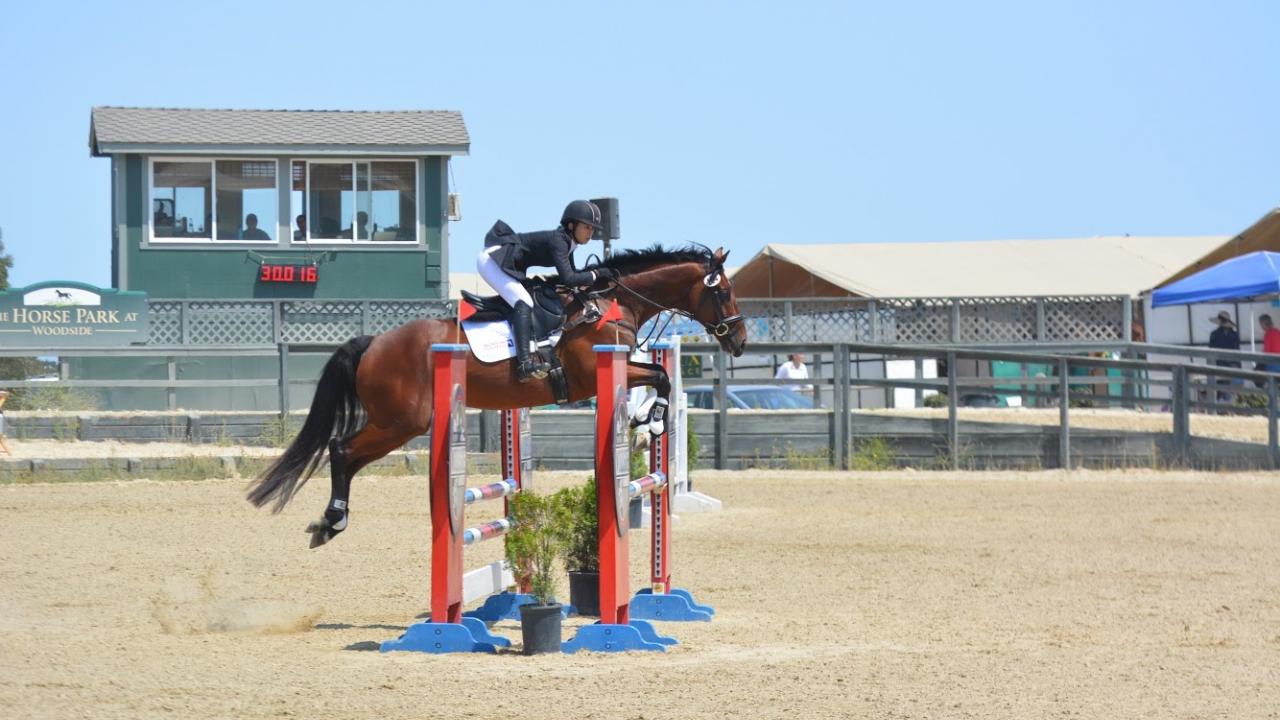The photograph captures a dynamic equestrian scene at the Horse Park at Woodside. A jockey, distinguished by a black helmet, black long-sleeved jacket, white pants, and black boots, is mid-jump on a dark brown horse with a black mane and tail. The horse is gracefully leaping over a red, white, and blue gate adorned with small flags. The clear light blue sky and sandy dirt track provide a picturesque backdrop. In the distance, a green grandstand with a few spectators is visible, along with a dark green booth equipped with a timer. A sign on the left of the image reads "Horse Park at Woodside," and nearby tents with beige triangular coverings add to the scene's charm. Beyond the main action, the rooftops of stables peek over the horizon, with some people picnicking under umbrellas, emphasizing the leisurely atmosphere of the practice session. The image radiates the elegance and intensity of equestrian sport, set against a serene outdoor venue.